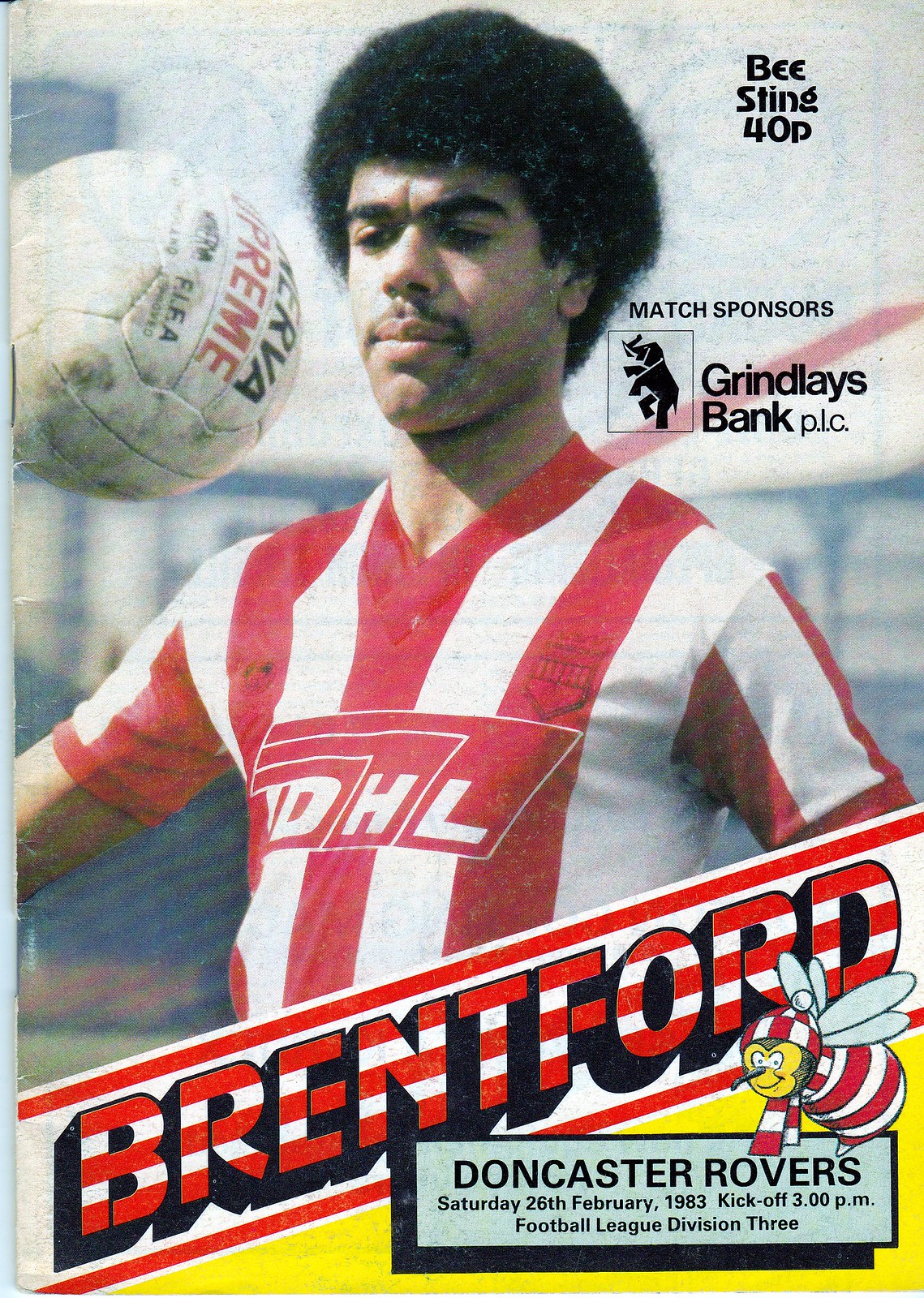This poster, advertising a Doncaster Rovers match, prominently features a soccer player with an afro positioned in the upper three-fourths of the image. The player, wearing a red and white vertically striped shirt with the DHL logo, is gazing at a white soccer ball near his face in the upper left corner. The ball has some partially readable text, including "RVA" and "Preme," though the rest is blurred. To the right of the player, the poster lists "Beesting 40P" and "Match Sponsors Grindley's Bank, P.L.C." An illustration of a bee dressed in a matching red and white striped sweater, scarf, and beanie appears below the player. The bottom portion of the poster includes a light blue text box with key event details: "Doncaster Rovers, Saturday, 26 February 1983, kickoff 3 p.m., Football League Division 3." The name "Brent Ford" in bold, striped text with a black drop shadow appears between two diagonal red lines in the bottom right quadrant, enhancing the overall design.